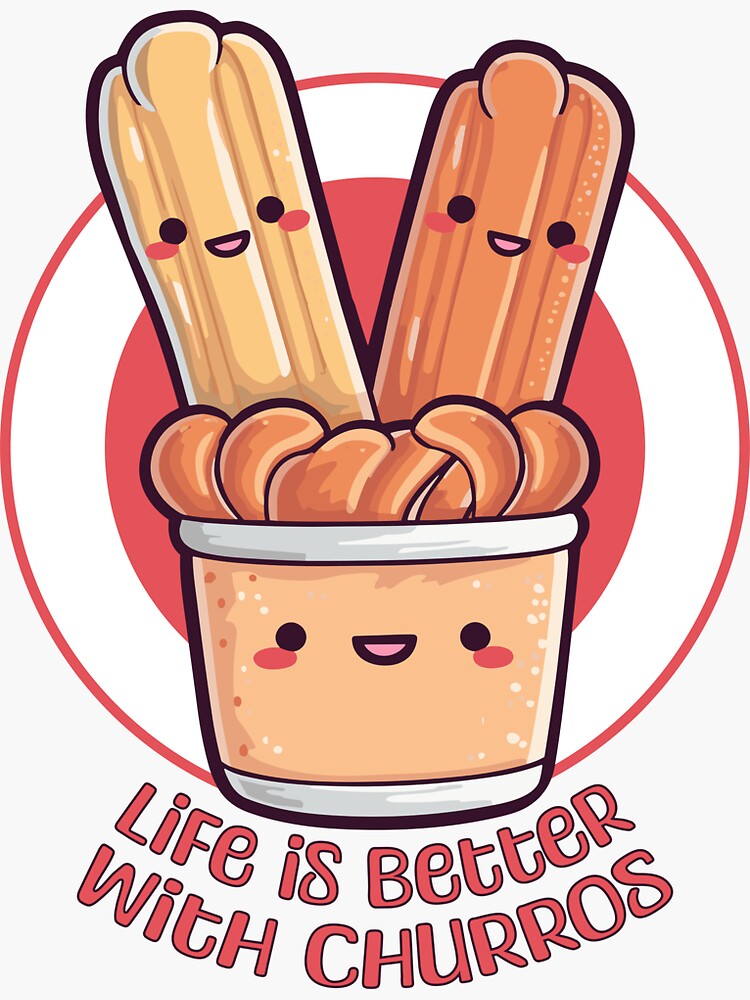The image is a cute cartoon drawing on a poster-like design, featuring two churros with happy, blushing faces coming out of a rounded cup that also has a smiling, blushing face. The cup is light orange with white borders at the top and bottom. The churros inside the cup appear in shades of blonde and golden brown, with some liquid-like waves of brown chocolate swirling around them. The entire drawing is set against a composition that looks like a target, with a light red inner circle and a larger outer border of pink. Below the cup, in pink text with a black outline curving along the bottom of the circle, the caption reads: "Life is better with churros."